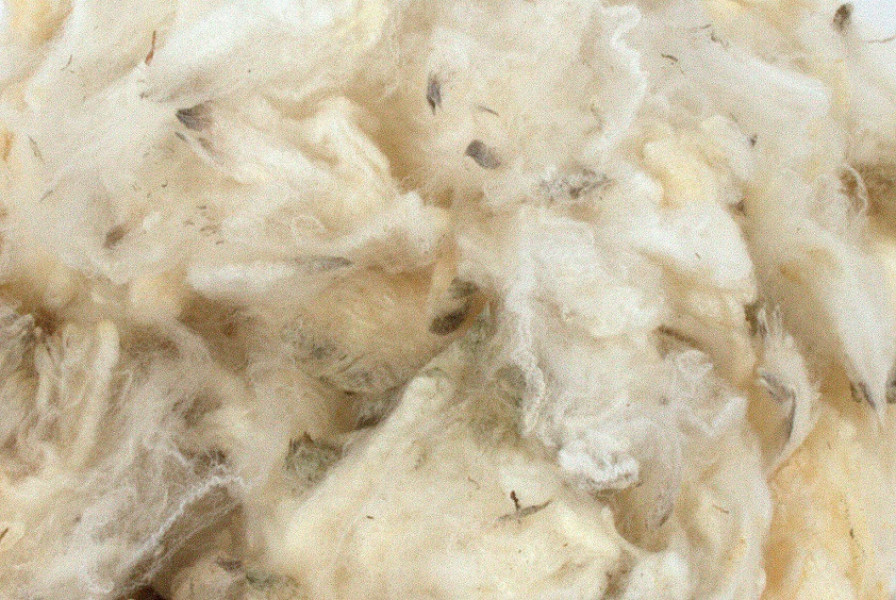This image is a detailed, close-up photograph of unrefined wool, possibly freshly sheared from a sheep. The wool predominantly displays a light cream color with some yellowish tints, indicating its natural, unprocessed state. Scattered throughout the wool are darker debris, including specks of brown, black, and gray, which could be dirt, seeds, or small pieces of plant matter. These impurities contribute to the wool's shaggy and uncombed appearance. The texture of the wool ranges from fluffy and soft in some areas to matted and clumped in others, giving it a varied and slightly crunchy feel. The wool fibers exhibit different forms, including stringy, zigzag patterns that highlight its rawness. There is no background visible in the photograph, as the wool fills the entire frame, and the image is well-lit, potentially using natural sunlight or bright indoor lighting. The intricacies of the wool and the uneven distribution of debris enhance the natural, untouched essence of the material.